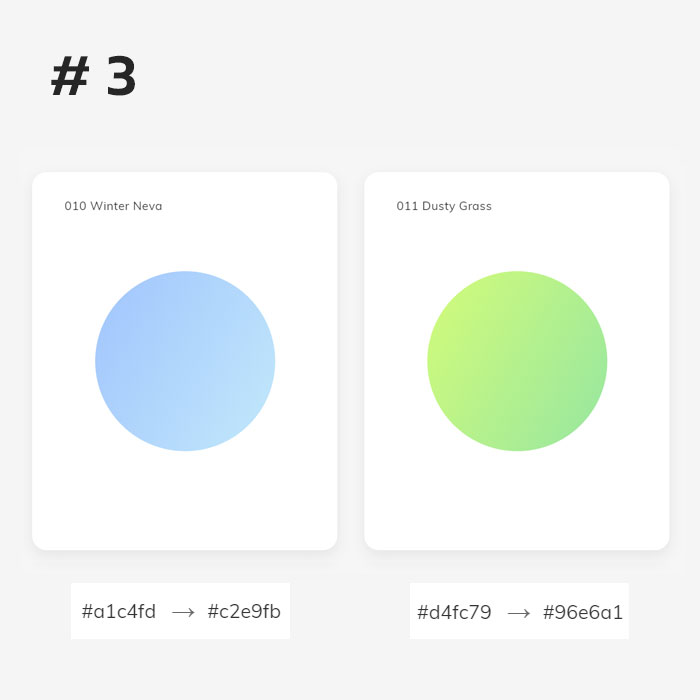This image features a light gray background with black text. On the left side, a bold black number "3" is prominently displayed. Directly beneath the number is a white square with text in the top-left corner that reads "010 Winter Niva" in black font. Centered within this square is a blue circle.

Adjacent to this square, there is another white box. Inside it, "011 Dusty Grass" is written in the top-left corner in black font, and directly below this text is a green circle.

Below the blue circle from the first square, there’s a sequence of text and graphics: a white box containing the black font "A1C4FD" followed by a gray arrow pointing to the right, leading to the text "C2E9FB."

To the right of this configuration is another white box with the text "#D4FC79" in black font, accompanied by a gray arrow pointing to the right, leading to another text "96E6A1."

All these elements are enclosed within a final gray box that borders the entire layout, adding a cohesive frame to the image’s composition.